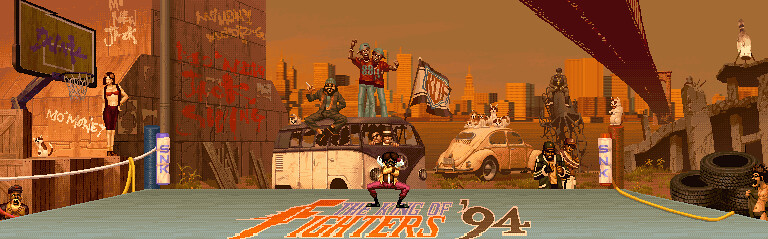This image appears to be a screen capture from a vintage video game, specifically "The King of Fighters '94." The background features an urban skyline indicative of New York City, including familiar landmarks like the Empire State Building and the Twin Towers, situating this scene firmly before the towers' fall. The skyline is rendered in shades of grayish tones, with an overarching red bridge stretching vertically on the right side. 

In the foreground, there's a blue fighting ring with rope boundaries, displaying "The King of Fighters '94" in vibrant purple, orange, red, and brown text. The ring is set within a basketball court under a bridge. A wall nearby is adorned with graffiti, adding to the gritty urban ambiance. On the left-hand side of the image, there's a basketball hoop also covered with graffiti.

The scene is populated with multiple characters: one central figure in a fighting pose at the center of the ring, dressed in pink pants and a yellow shirt. Surrounding the ring are spectators, including a man and woman on the left, a person squatting on the court, and two individuals in blue pants, red shirts, and blue hats standing atop an old van. Additional spectators can be seen through the van’s windows and perched on its roof. Alongside these figures, various other individuals, including a cat on a pole, add to the rich detailing of the scene. The overall color scheme leans towards hazy shades of tan and orange, reinforcing the vintage and retro video game aesthetic.